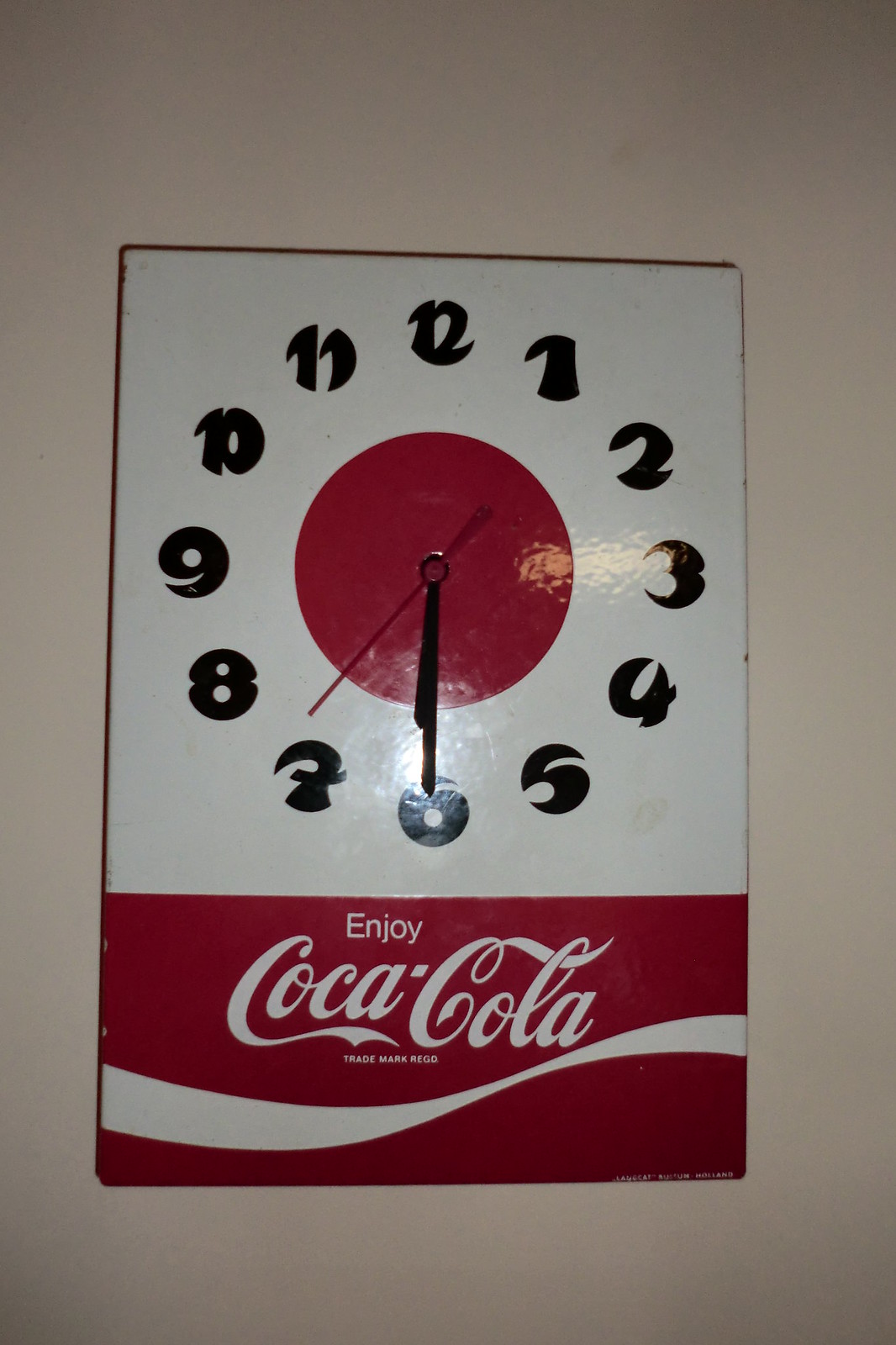This photograph features a rectangular clock mounted on a beige wall, prominently centered in the frame. The clock's design is striking, with the upper two-thirds of its face displaying a pristine white background dominated by a large, solid red circle at the center. The timepiece is equipped with bold black hour and minute hands, complemented by a vibrant red second hand. Its numbers are distinctively thick and end with a curvy flourish, adding a touch of whimsy to the otherwise modern design. The time on the clock is set to 6:30.

The lower third of the photograph transitions to a bold red background. At the top of this section, centrally aligned, the word "enjoy" is inscribed in small white letters. Directly below it, also centered but in larger white text, is the iconic "Coca-Cola" logo, rendered in its classic cursive script. Beneath the logo, the signature white wavy ribbon associated with the Coca-Cola brand completes the design, enhancing the cohesive and nostalgic feel of this visually appealing image.